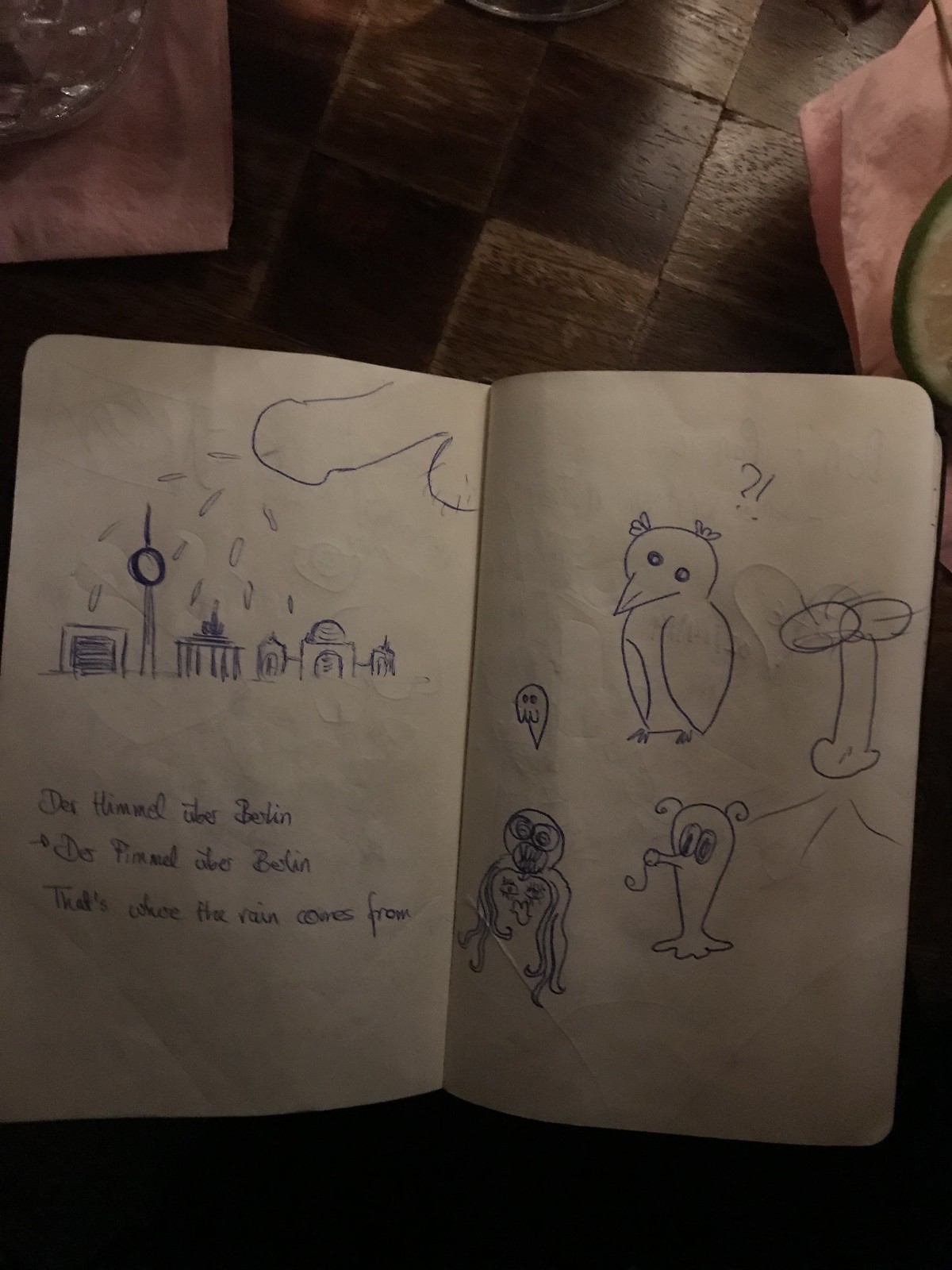In the image, a small white notebook rests atop a brick floor composed of various shades of brown bricks. In the background, a red cloth can be seen partially, holding what appears to be a bowl of items, alongside another red cloth and the edge of an unidentified object. The notebook is open to two pages filled with intricate drawings. On the left page, there is a detailed illustration of a quaint town under a big, billowing cloud from which rain pours down onto the buildings below. The right page features pencil sketches of small animals, including what appears to be an owl or a bird at the top, and a whimsical, little monster at the bottom. The scene combines elements of art and a cozy setting, providing a charming glimpse into a moment of creative expression.